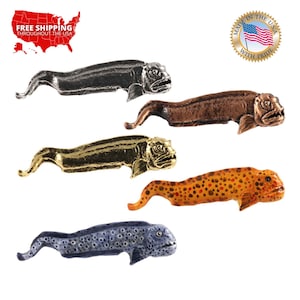The image displays a detailed arrangement of small eel-like sculptures lined up in two columns against a white background. In the upper left corner, there's an icon of the United States shaded in red, including Hawaii, with white letters that read "Free Shipping through the USA." Additionally, there's a seal in the upper right corner – a gold circle encasing an American flag with "Made in the USA" inscribed around it.

Five distinct sculptures, seemingly crafted from blown ceramic or metal, are aligned vertically. From top to bottom, the left column features a dark gray and silver eel, a gold eel, and a blue patterned eel with black polka dots. To the right, there's a bronze eel followed by an orange eel with black polka dots. Each sculpture depicts an open mouth with visible teeth, a single fin on the front, and a continuous tail with no back fins, contributing to their quirky and somewhat ugly appearance.